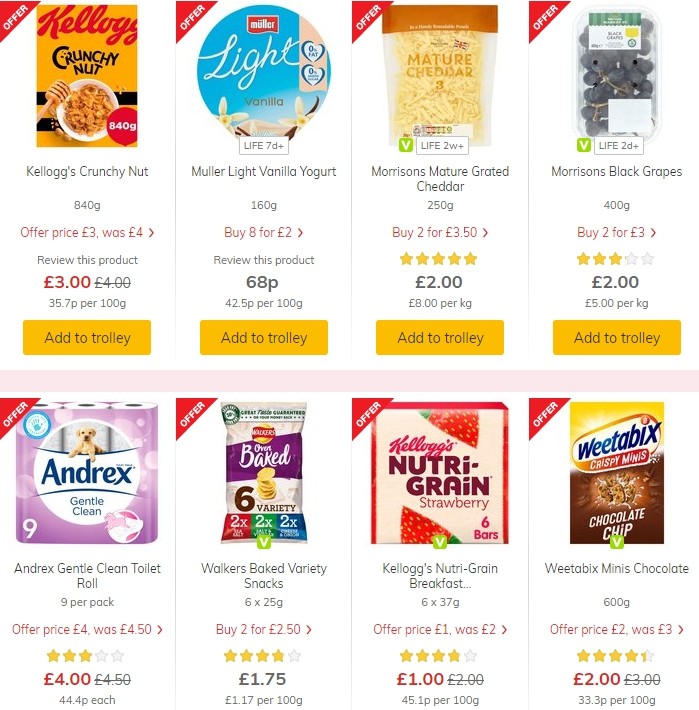This screenshot features a clean, white background. At the top, it showcases four vertical product listings, each marked by a red triangle in the upper left-hand corner with the word "Offer" written diagonally in white text. Adjacent to these triangles are images of the featured products. The first product is a box of Kellogg's Crunchy Nut cereal. Beneath the image, the name "Kellogg's Crunchy Nut" is printed in small black text. Below the product name, "Offer Price" is displayed in a pale red font, followed by "Review This Product" written in black. The actual price of the product is prominently shown in red, and at the bottom of each listing is a yellow "Add to Trolley" button.

A thick light pink horizontal line separates these top listings from a lower row of four more product entries. However, these bottom entries are partially cut off by the screenshot's edge, obscuring the "Add to Trolley" button for each. Some products include a star rating above the price. These ratings feature yellow stars; unselected stars appear gray. When a product does not have a rating, the "Review This Product" text is displayed instead.